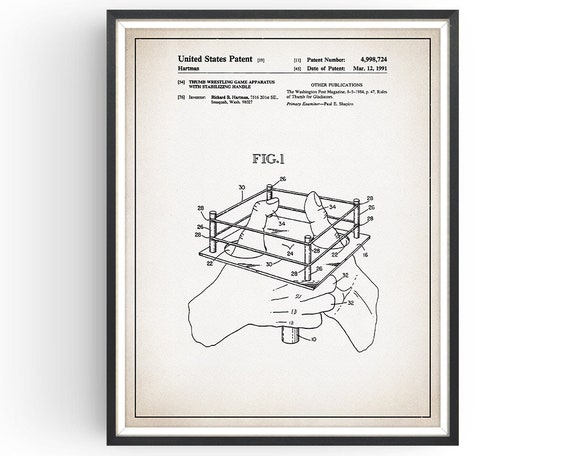The image depicts an aged, black-framed print set against a white background. The frame is thin with a black wood finish, surrounding an 8x11 styled print that features a thin white border. The central image and text are in a brownish-grey hue, giving it an old-fashioned appearance. At the top, in bold black text, it reads "United States Patent," with "Hartman" noted on the left side, although slightly obscured. To the right, it provides the patent number "4,999,724" and the date "March 12, 1991." Below this, text describes a "wrestling game apparatus." The illustration portrays two thumbs engaged in a thumb wrestling match inside what looks like a miniature wrestling ring, complete with ropes. The image hints at a toy designed for thumb wrestling, capturing a blend of technical schematics and playful design.